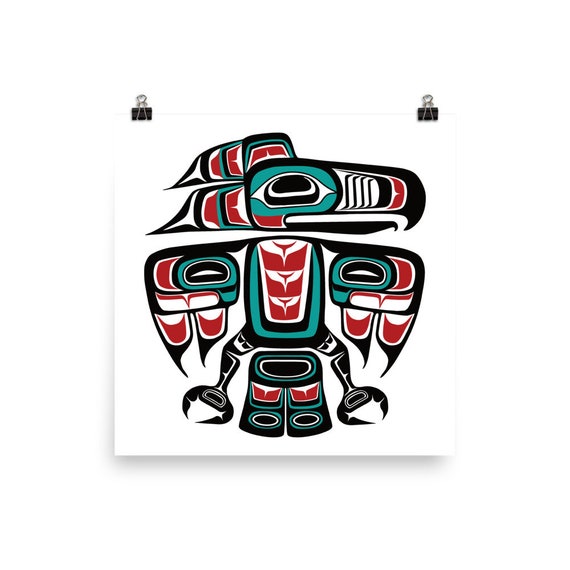The image showcases a color photograph of a square-format art print done in the Pacific Northwest Haida native style. The artwork, depicted on a white canvas suspended against a white wall using black paper binding clips at the top left and right corners, features a vibrant tribal representation of a raven. The raven's head is turned to the right, showcasing a large, curved black beak and a prominent eye encircled by blue. Red feather shapes adorn the top and back of the head. Thick black lines delineate the intricate design, with bold colors of blue, green, red, white, and black enhancing the visual impact. The raven's symmetrical body faces the viewer, with wide-spread wings that transition from aqua at their centers to red feathers towards the tips. The bird stands on its black tail feathers, with its two feet pointing to the right. The overall aesthetic combines traditional indigenous artistry with a modern photographic color illustration, emphasizing the bold and striking characteristics of Haida raven art.